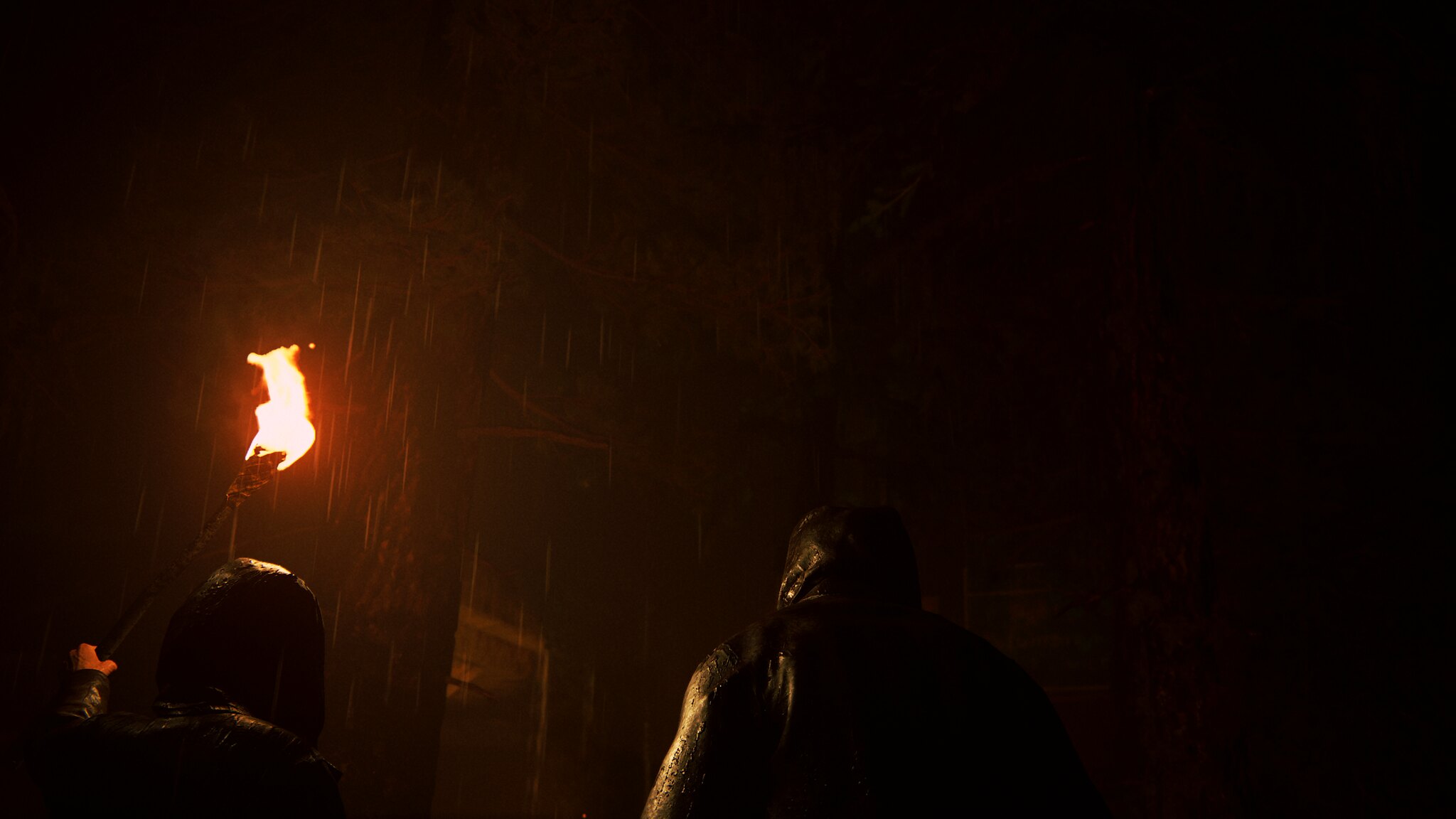The image is rectangular, characterized by a predominantly dark and blurred ambiance with limited clarity and detail. Despite the poor quality, the outlines of two individuals are discernible. The first person is positioned on the bottom left, holding a torch aloft in their left hand. The torch emits white and orange flames that contrast against the darkness. They are dressed in a black hoodie, enhancing the silhouette effect against the ambient shadow. The second individual stands towards the bottom center, also clad in a black hoodie and jacket. The rest of the image fades into near-total darkness, creating a stark and mysterious scene.